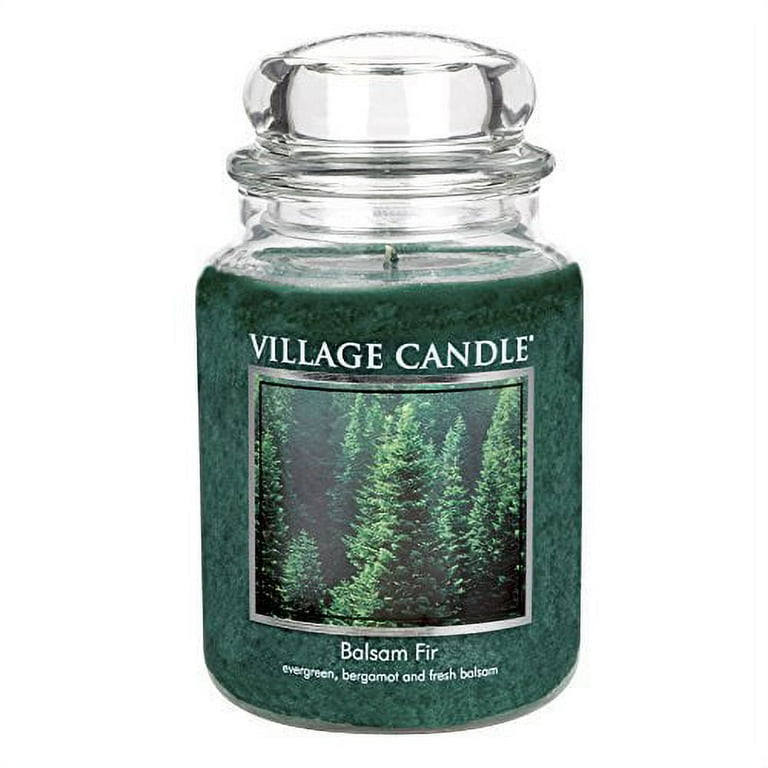The image showcases a large, dark green jar candle from Village Candle, housed in a clear glass jar with a matching rounded glass lid. The candle features a small white wick at the center and appears to be almost filled to the top, indicating it hasn't been lit yet. Prominently displayed in white, uppercase letters is the brand name, "Village Candle," followed by a square label depicting a forest of evergreen trees. Below the image, the candle's scent, "Balsam Fir," is written in white, along with smaller white text listing its aromatic notes: Evergreen, Bergamot, and Fresh Balsam. The overall design and presentation are similar to that of Yankee Candle products.